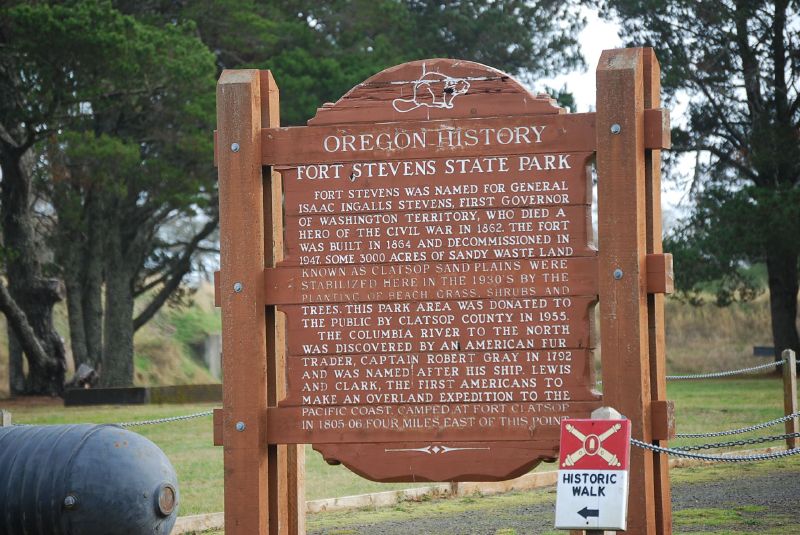The photograph captures a wooden historical marker at Fort Stevens State Park in Oregon. The sign, mounted on two wooden posts and adorned with a carved illustration of a beaver at the top, reads: "Oregon History Fort Stevens State Park." The text details that Fort Stevens was named after General Isaac Ingalls Stevens, the first governor of Washington Territory, who died heroically in the Civil War in 1862. The fort was constructed in 1864 and decommissioned in 1947. In the 1930s, around 3,000 acres of the Klatsop Sand Plains were stabilized with beach grass, shrubs, and trees, and the parkland was handed over to the public by Klatsop County in 1955. Further historical notes include the discovery of the Columbia River by Captain Robert Gray in 1792 and the Lewis and Clark expedition’s camping at Fort Klatsop in 1805-06, just four miles east. Below this panel is a smaller sign with a red symbol, cross swords, and the words "Historic Walk," pointing left. The wooden marker is bordered by a chain-link fence, with trees and grasslands in the verdant background. To the lower left of the image, there is the rear of a cannon visible, adding a historic military touch to the scene.